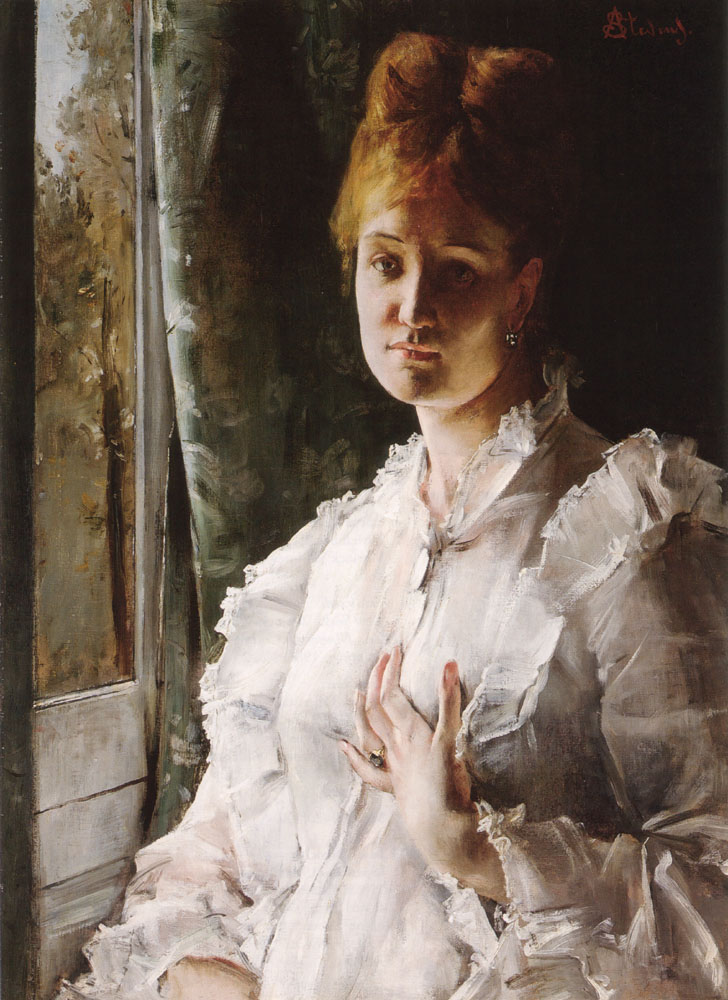The painting depicts a despondent-looking woman with reddish-brown hair, styled in an updo with a poofy top and part in the center. She wears a frilly white blouse and a gold wedding ring with a dark emerald stone. Her right hand rests over her chest while her other hand lies over her stomach. An earring adorns her visible ear. The backdrop features a green curtain with a floral pattern and a window, through which lush greenery in light green hues and a faded white wall can be seen. The artist's signature, possibly reading "Atwing," is located in the top right corner of the painting.